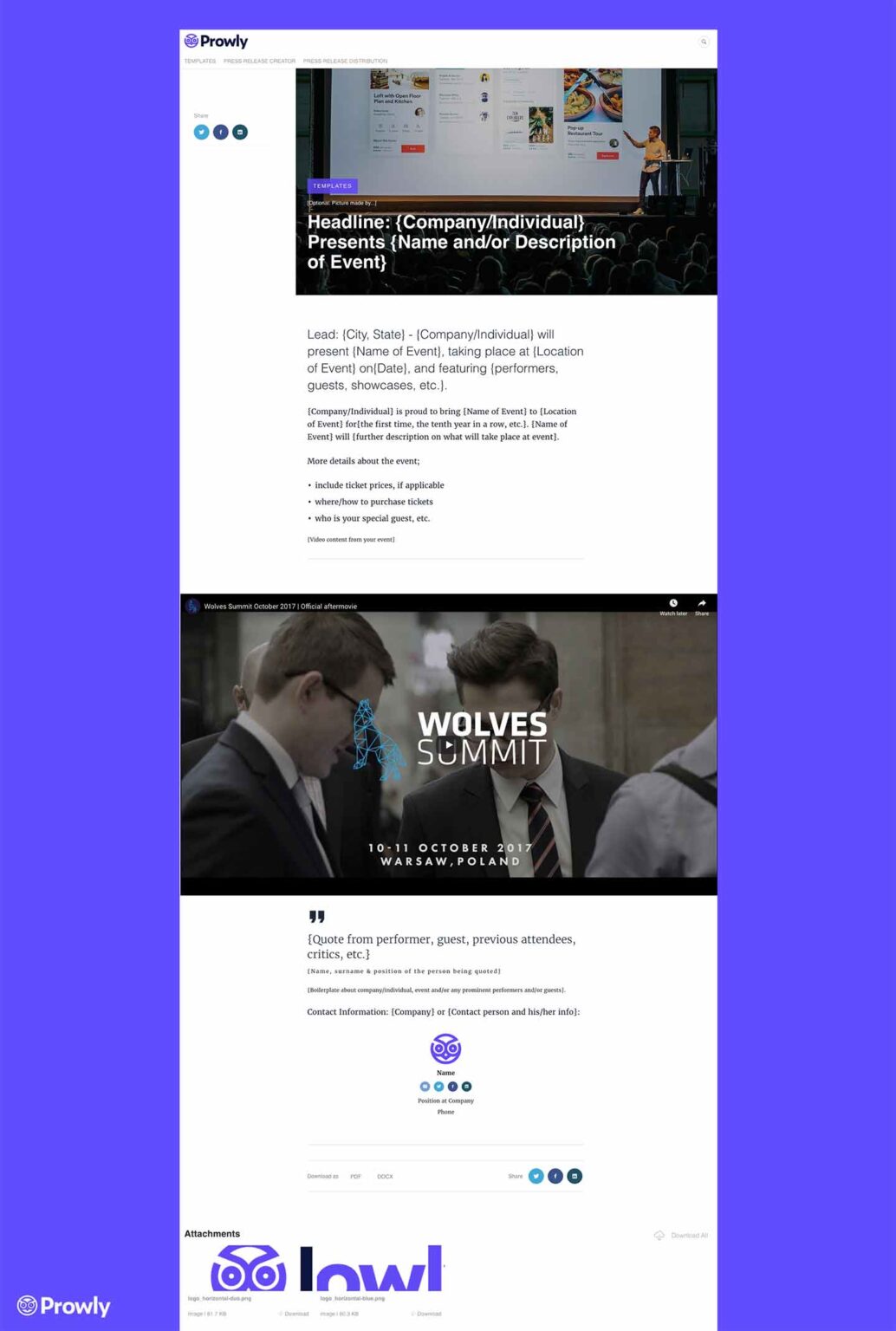**Caption:**

The image depicts a vertical-oriented webpage with various design elements and text sections. 

- **Background and Perimeter:** The main content is framed against a purple background on the left, right, and a small portion at the top. A white logo with "Prowley" in white letters is positioned in the lower left corner.

- **Header:** At the very top, there's a long white bar featuring a purple logo followed by "Prowley" in black letters. Below are three gray, unidentifiable menu options.

- **Main Content Area:**
  - **Left Section:** Dominated by a large white area containing a small gray word towards the top (indistinguishable), followed by three icons (one light blue and two dark blue), and an unexplained white dot in the middle.
  - **Right Section:** Contains a rectangular image of a Caucasian male in a yellow shirt, pointing at a screen with multiple website options. The foreground features silhouettes of an audience. A blue rectangular button with unreadable white text is to the center-left of this image.
  - **Text Details:** Below the image, in white letters, are the words "headline: (company, individual)," followed by "presents [name and/or description of the event]." There are two paragraphs in black text, followed by a sentence comprising three black bullet points, and additional small, unreadable black text.

- **Embedded Image/Video:** A lower section features an image of two Caucasian men in business suits with short black hair. Overlaying the image is a blue wolf icon. To the right, white text reads "Wolf Summit" with a play button in the center. Beneath this, it states "10-11 October 2017 Warsaw Poland," indicating a playable video. 

- **Footer and Additional Elements:**
  - Left of this section is black text that likely reads "advertisement(s)." Surrounding the text are icons: a purple owl logo underneath some faint gray text, and further unreadable gray options. 
  - Right of the playable video icon are further gray and blue elements: gray text (too small to read), light blue text boxes with light dots, dark blue circles with white dots. 
  - At the very bottom, black letters are mostly legible spelling out "advertisement(s)" and an owl logo in purple, but this is truncated by a black bar with remaining gray text that is too small to discern.

The overall design suggests a high-level summary of an event, person, or company, presented within a complex webpage layout.